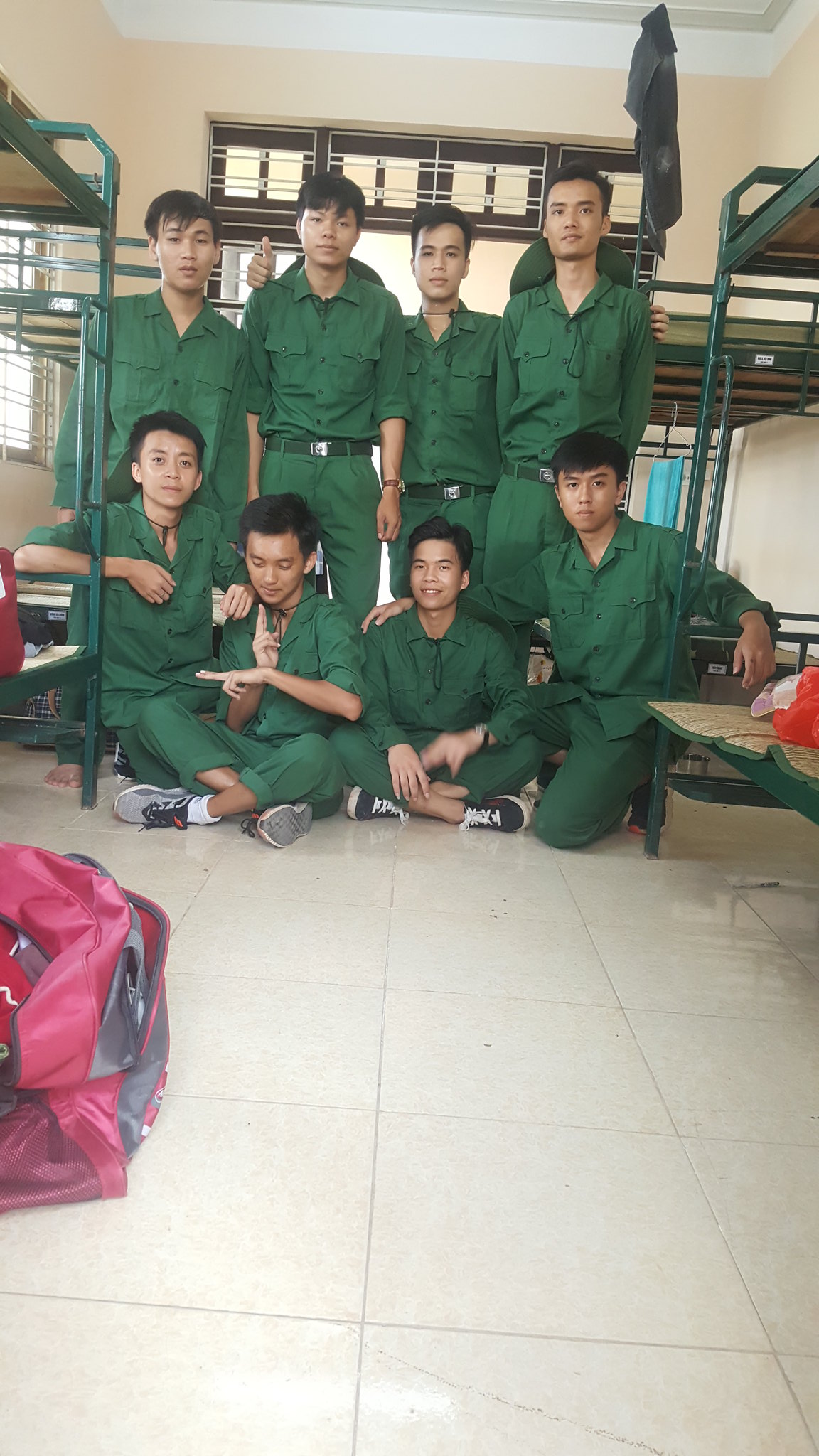This image appears to be taken inside a military barracks or jail-like facility during daylight hours, as indicated by the light streaming through barred windows. The floor is made of white tiles, and the walls are painted cream, contrasting with the white ceiling. Prominently, a red duffel bag sits on the floor in the foreground, with another red bag positioned on a bunk bed in the background. The room features green-painted wooden bunk beds with minimal padding rather than full mattresses.

At the center of the image, eight men of East or Southeast Asian descent, likely military personnel in green uniforms, are posing for the photograph. The group is divided, with four men standing and the other four sitting or kneeling on the tiled floor. They are positioned between two rows of bunk beds with green metal frames. The men are closely grouped, some with their arms around each other, displaying a range of expressions from slight smiles to neutral looks. One man, who is sitting cross-legged on the floor, stands out with a wide smile, adding a subtle touch of warmth to the otherwise stark setting.